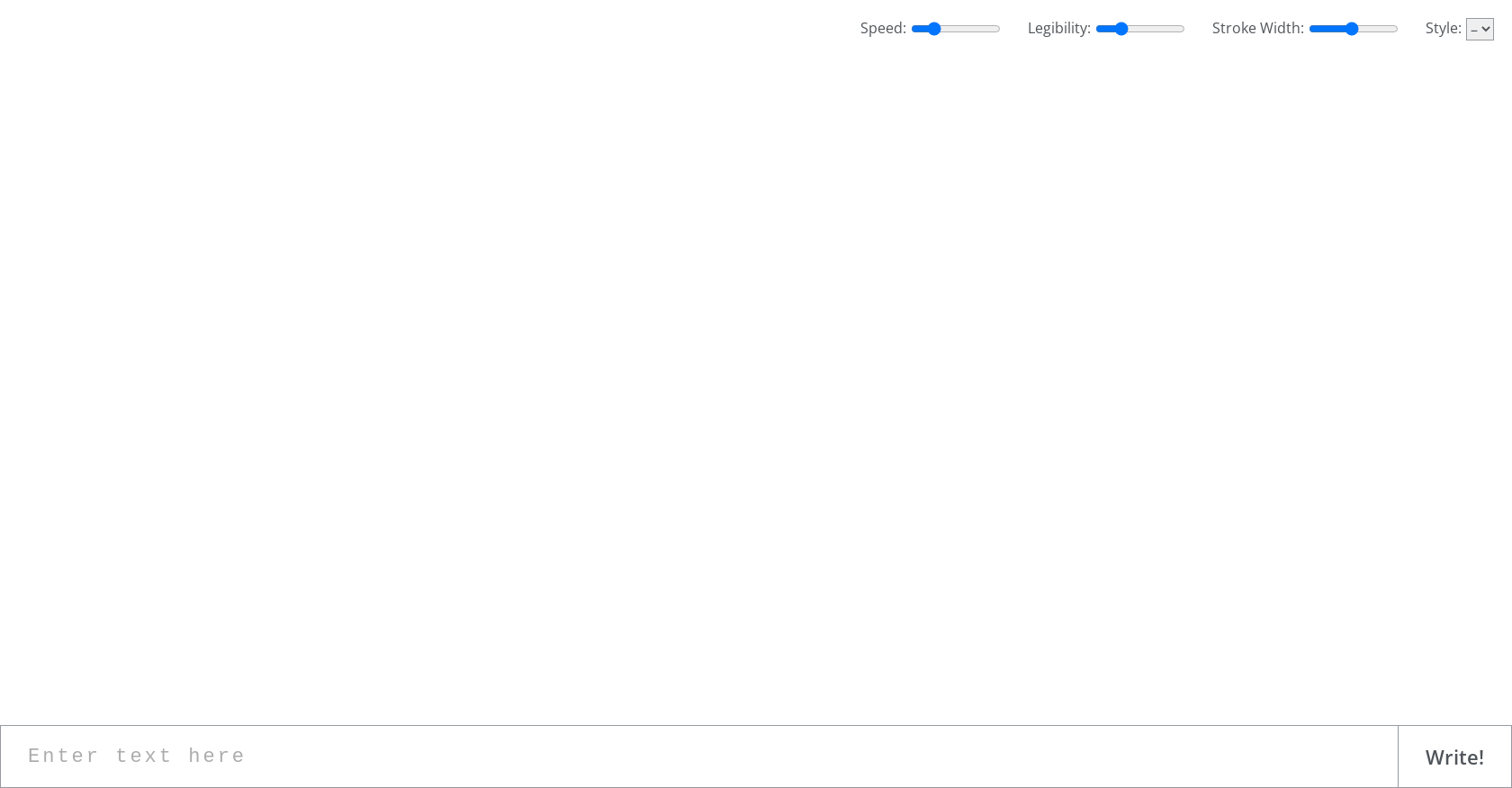The image depicts a screenshot of a user interface, possibly for a web application or a mobile app. The primary content area is a blank white page, but there are notable elements at the top and bottom of the screen.

**Top Section:**
- On the right side, three adjustable sliders are present:
  1. **Speed:** A gray bar with a small portion in blue, indicating its adjustable level. It appears similar to a typical slider bar used for setting values, possibly to indicate percentage or intensity.
  2. **Legibility:** Another slider bar that is mostly gray, with a small segment in blue, suggesting it's set to a low level.
  3. **Stroke Width:** This slider is balanced with half of the bar in blue and half in gray, suggesting a mid-level setting.

Each of these sliders features a small circle in the middle, indicative of the draggable portion for adjusting the values. At the far right end of this section, there's a drop-down menu labeled "Style".

**Bottom Section:**
- A text/search box is located at the bottom of the page. It contains a placeholder text that reads, "Enter text here".
- Next to this box, there is a button labeled "Write".

The interface appears minimalistic and functional, likely designed for a specific task involving text input and adjustments to visual settings like speed, legibility, and stroke width.